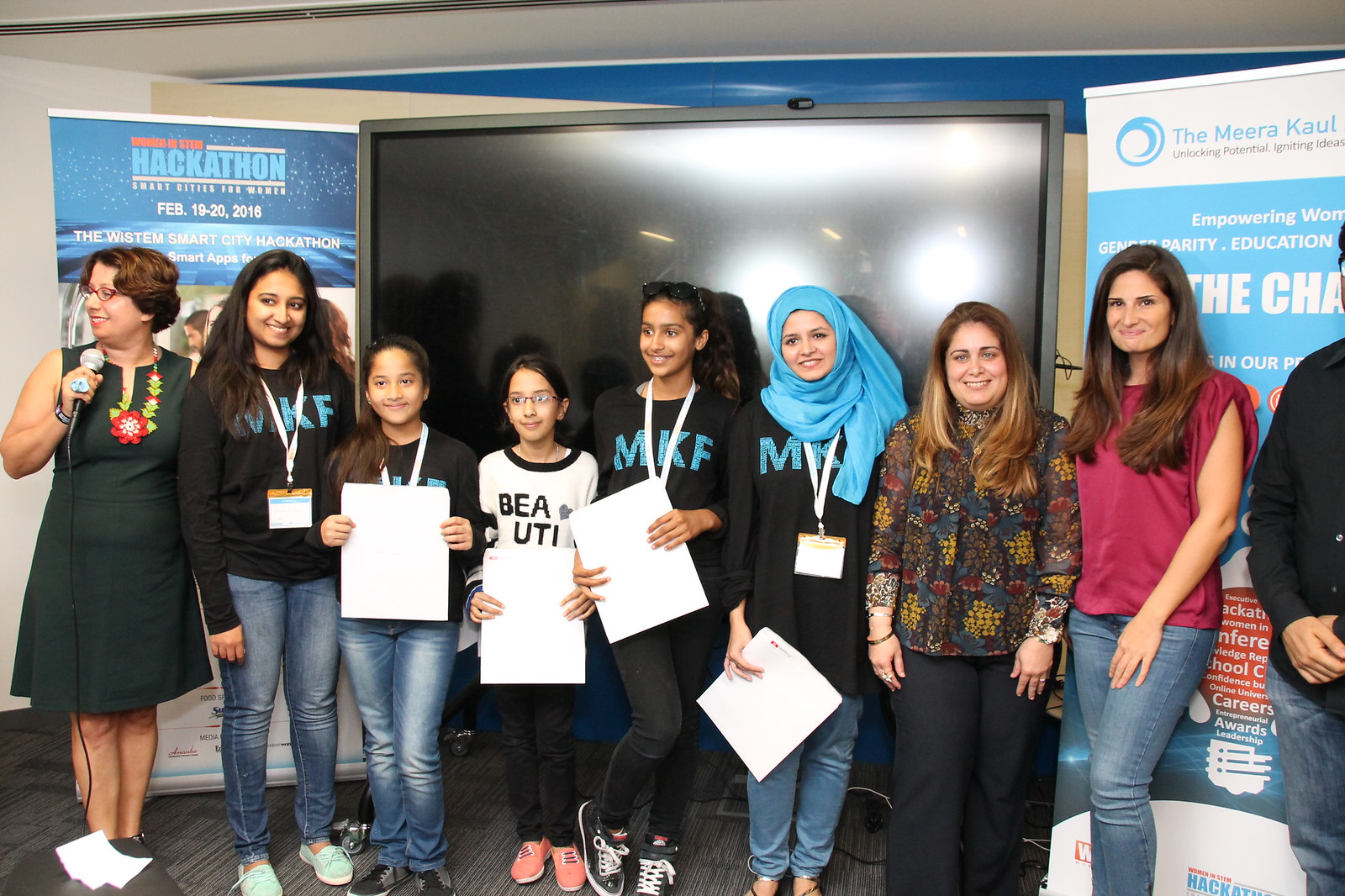The image depicts a group of young girls and women standing in a line in front of a large black screen. They are flanked by two tall standing posters on either side. On the left, a woman with short brown hair and wearing a dark green dress with a rose or red petal on her chest holds a microphone and looks to the left. Another woman next to her wears a black dress with red glasses and appears to be addressing the group. 

A girl next to her wears a shirt saying "MKF" on a black background and blue jeans. Following her, another girl also in an "MKF" shirt and blue jeans stands with a large piece of paper. Then, a young girl smiling and wearing sunglasses holds her piece of paper diagonally, while the next girl in the row, wearing a white t-shirt and glasses, holds a large paper rectangularly. 

Further to the right, a woman in a blue headscarf and an "MKF" shirt smiles brightly, holding a piece of paper by her side. Another woman with brown hair and a patterned shirt and trousers smiles as well. Next to her stands a taller woman in a red shirt, black jeans, and holding another piece of paper. It ends with a man in a black shirt and blue jeans, standing with his hands clasped and also holding a microphone.

The background features a blue and white ceiling and a black wall with a screen turned off. The left poster reads: "Women in STEM Hackathon, Smart Cities for Women, Feb 19-20, 2016. The Wisdom Smart City Hackathon, smart apps." The right poster highlights: "Unlocking potential, uniting ideas, empowering women, gender parity education," along with a mention of a powerful empowering women's event. The space also includes text too small to read in the provided details. 

Overall, the scene represents a diverse group of young women and an inclusive event centered around women in STEM and empowering women through education and smart city innovations.